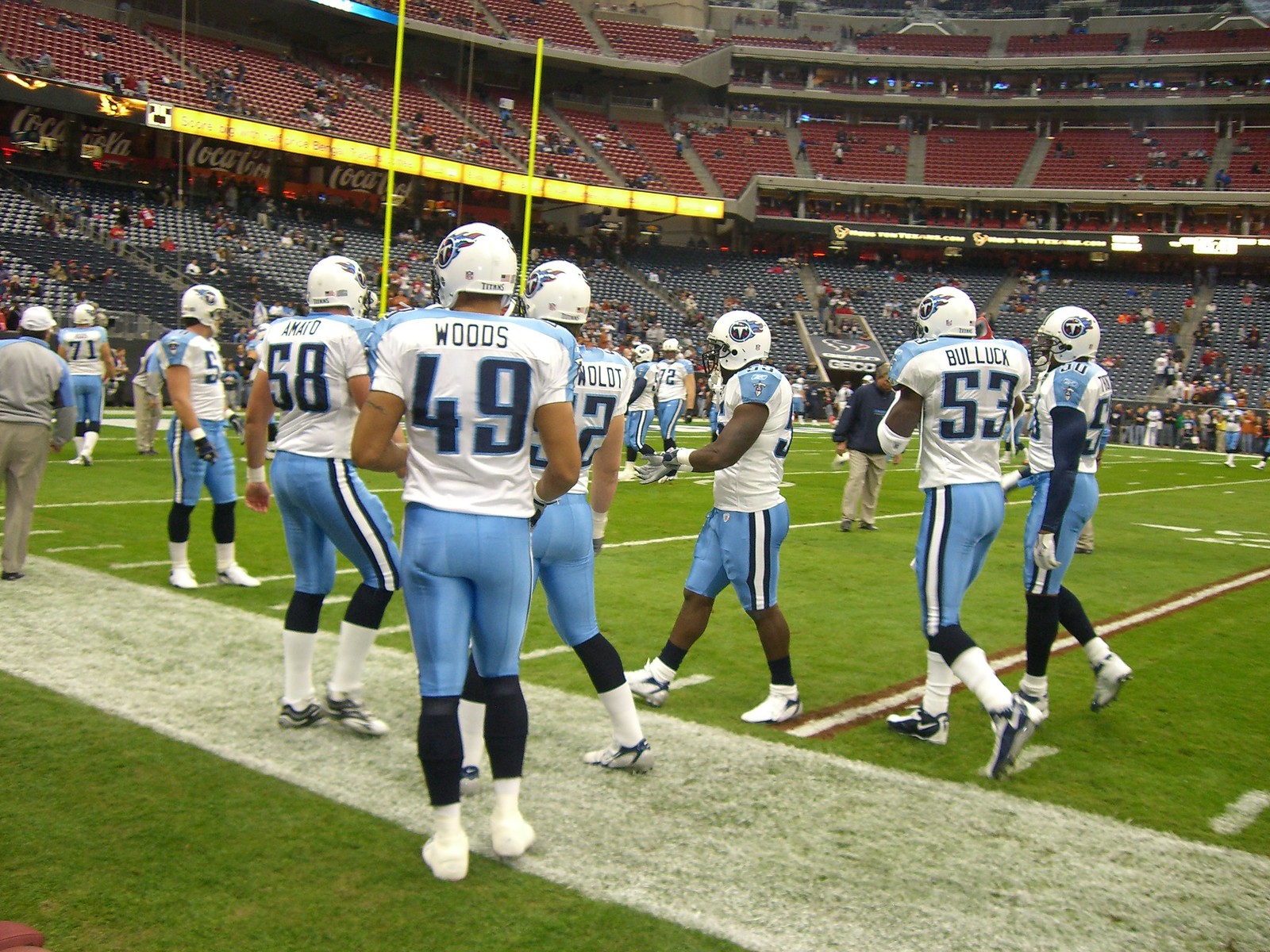A detailed, cleaned-up caption:

"The image showcases an expansive, flat grass field with clearly painted lines, indicative of a football stadium. The field is adorned with various vividly colored markings. At the top of the image, rows upon rows of empty seating hint at a largely unoccupied stadium. In the center of the frame, football players stand prominently, their jerseys displaying their names. The scene is bathed in an array of colors, including green, brown, white, light blue, dark blue, red, and yellow, all under the canopy of a nighttime sky. This outdoor setting, characterized by the distinct layout and ambiance of a football stadium, captures a serene moment before or after a match."